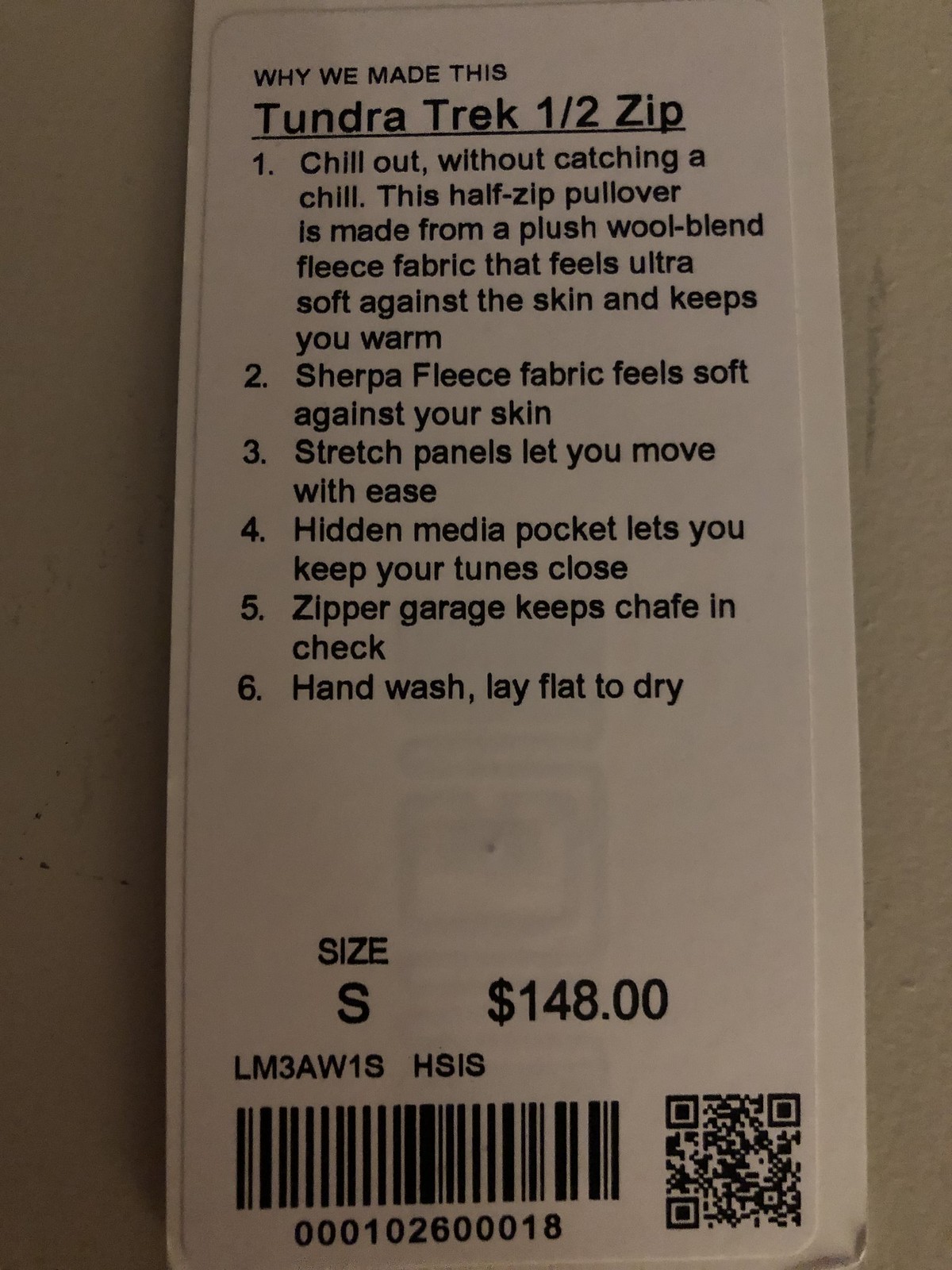This image is a close-up of a white care tag against a painted white wall background. The tag provides detailed information about a clothing item named, in bold and underlined black letters, "Tundra Trek Half Zip." The top of the tag features the phrase "why we made this," followed by a numbered list of six detailed points about the garment. 

1. The first point states, "Chill out without catching a chill. This half zip pullover is made from a plush wool blend fleece fabric that feels ultra soft against the skin and keeps you warm."
2. The second point highlights that the Sherpa fleece fabric adds to the softness against the skin.
3. A further feature includes stretch panels for ease of movement.
4. The fourth point describes a hidden media pocket for keeping personal audio devices close.
5. The fifth point mentions a zipper garage to prevent chafing.
6. The final point instructs the owner to hand wash the garment and lay it flat to dry.

At the bottom left of the tag, the size is noted as "S" for small, and to the right, the price is marked at $148. The lower part of the tag includes a barcode, a QR code, and additional product codes for inventory.